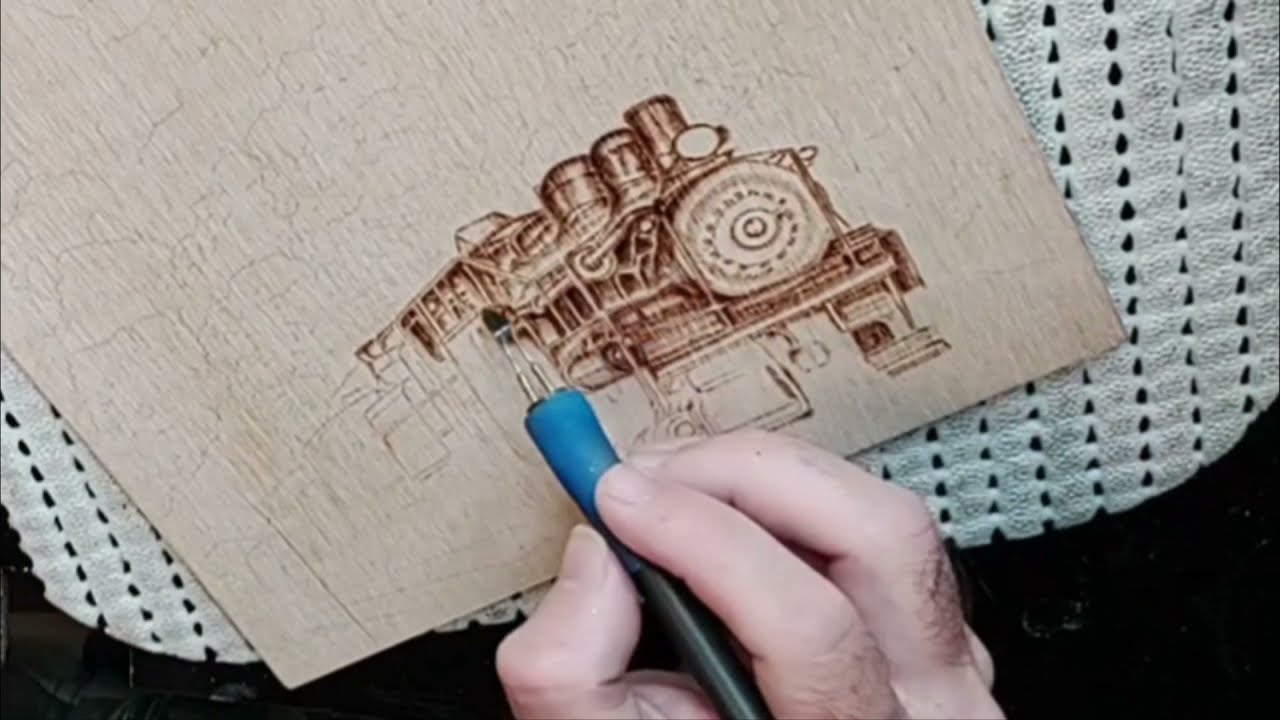The image captures a detailed scene of an intricate hand-drawn train being carved onto a piece of brown wood. The train’s engine, complete with visible smokestacks, is meticulously outlined and shaded, suggesting an advanced stage of the artistic process. A person's hand, lightly tanned with visible hair on the fingers, is seen gripping a specialized tool. This tool, featuring a black base and a blue tip, appears to be equipped with twin metal forks used for carving or burning the design into the wood. The wood itself rests on a white, perforated fabric, which is draped over a black surface, possibly a table or a counter. This setup provides a stark contrast, highlighting the intricate details of both the artwork and the crafting process.